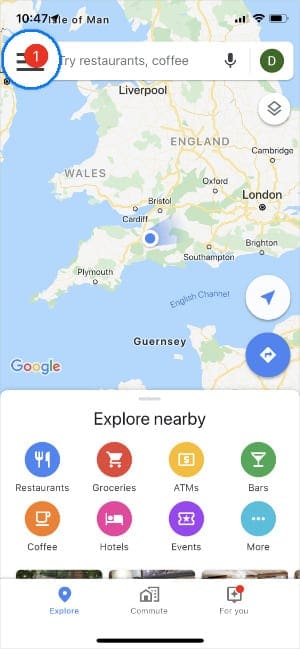The image depicts a smartphone screen with various elements. The status bar at the top shows the time as 10:47, a strong Wi-Fi signal, and a nearly full battery. Below the status bar, there is handwritten text mentioning "Red Circle, 1, train rations, coffee, a microphone, D". 

The background of the phone screen appears to be a map of the United Kingdom, highlighting cities such as Liverpool, Wales, Plymouth, Bristol, Oxford, London, Brighton, Southampton, and Cambridge. The map also shows features such as the English Channel and the island of Guernsey. 

At the bottom, there's a navigation panel on a blue backdrop, with icons indicating various categories such as a knife and fork for restaurants, a grocery cart for groceries, and an ATM for cash withdrawals. There are colored circles for different amenities: 
- Red circles denote grocery stores
- Yellow circles represent ATMs
- Orange circles signify coffee shops
- Purple circles indicate hotels
- Blue circles mark events

Below this navigation panel, the screen displays options labeled "Explore Nearby," "Explore," "Commute," and "For You," suggesting personalized recommendations for the user. The visual elements highlight several of England's cities and practical tools for exploration and daily tasks.